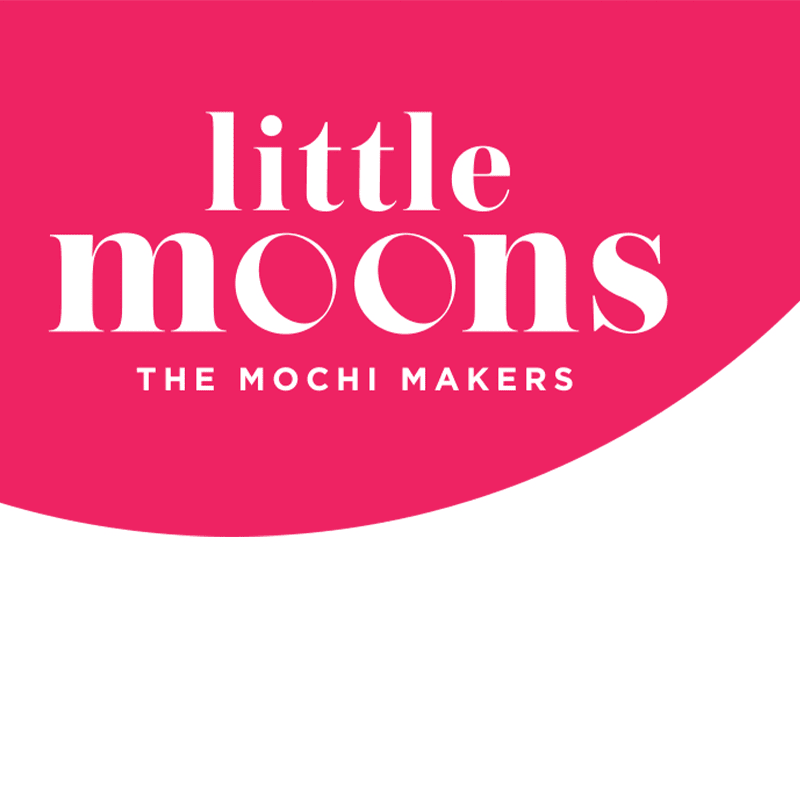The image is a company logo with a predominantly red and white color scheme, divided horizontally. The top section, which covers about three-quarters of the image, is red and features a downward arching line that extends from the lower left to the mid-right side. In this red portion, centered, the text reads "little moons" in lowercase white letters, with the "O"s stylized as crescent moons. Below this, in smaller, all-capital white letters, it says "THE MOCHI MAKERS." The remaining quarter at the bottom of the image is white. The entire design presents a modern and clean look, likely representing a brand associated with mochi, a traditional Japanese food.